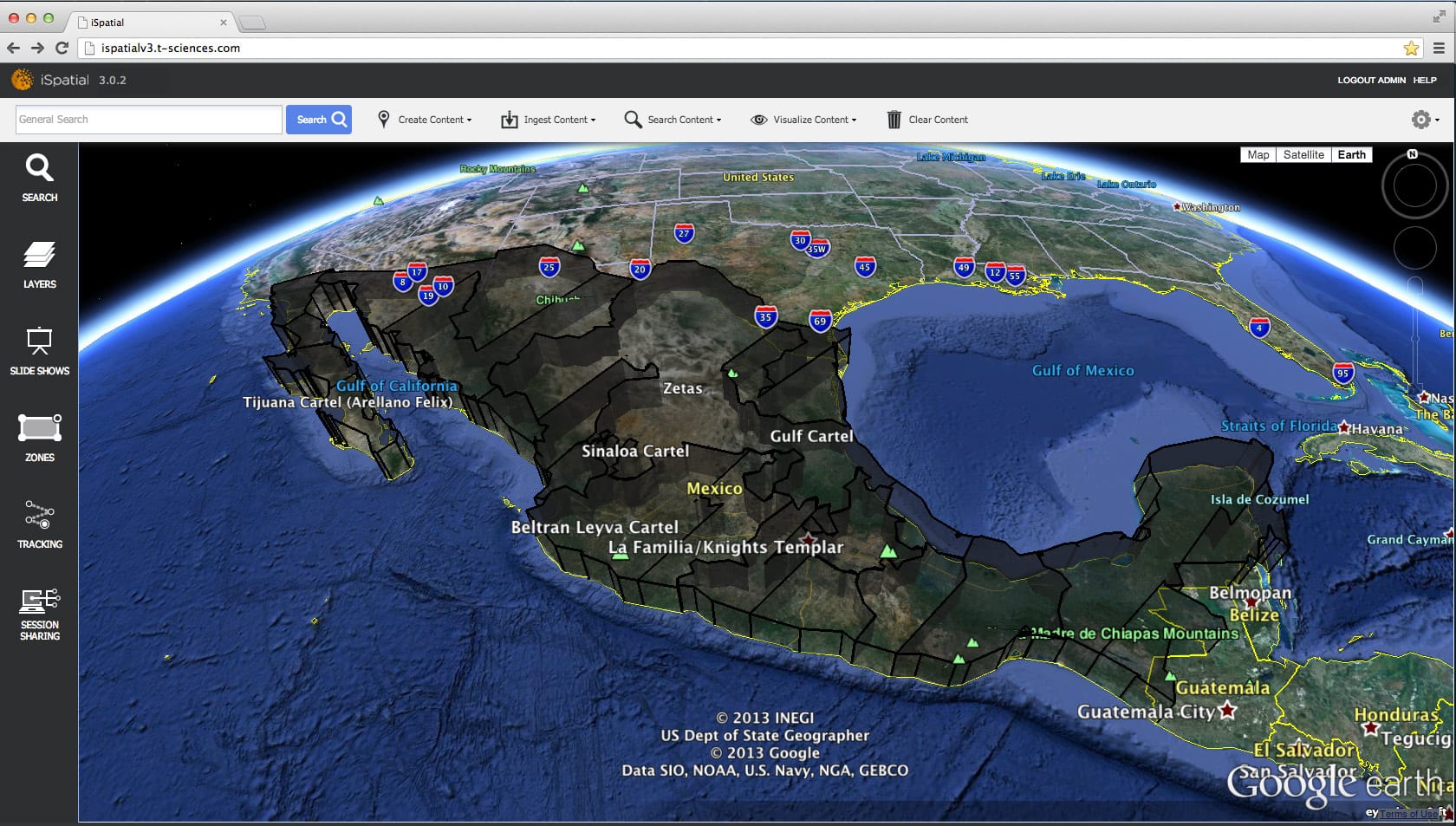This detailed screenshot portrays a map of the Earth viewed from space, prominently featuring North and Central America. The United States is positioned at the top, with the Gulf of Mexico clearly visible. In Mexico, various regions are labeled with the names of known drug cartels, including the Sinaloa Cartel, the Beltrán-Leyva Cartel, La Familia Michoacana, Knights Templar, Los Zetas, and the Tijuana Cartel. Additionally, the map highlights key geographical areas such as Guatemala, El Salvador, Belize, Honduras, and Cozumel. 

Distinct highways are marked with shield icons, primarily in Mexico, delineating the states. Green arrows traverse the map, potentially indicating drug trafficking routes, though this is not explicitly stated. The Gulf of California is also labeled, contributing to the map's geopolitical context. The map is credited to the U.S. Department of State Geographer, providing an official and authoritative source for the depicted information.